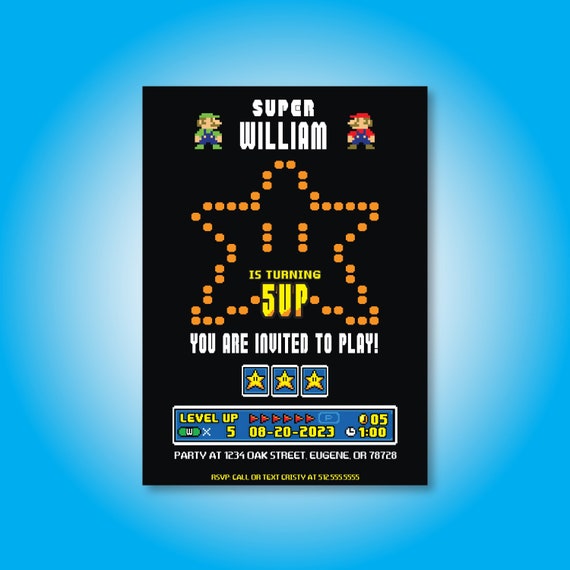The image features a vibrant blue background with a central black rectangle, reminiscent of a video game interface. At the top of the black rectangle, "Super William" is written in bold white letters, flanked by Luigi on the left and Mario on the right. In the middle, there is a star made out of orange dots, complete with dotted eyes, symbolizing the classic power-up from the Super Mario games. Below the star, in bright yellow text, it reads "is turning 5 up." Following that, in white text, it says, "You are invited to play."

Under this text, there are three yellow stars against a blue background with white borders, further emphasizing the gaming theme. Below the stars, another blue rectangle with a white border contains the text "level up." This section also displays several elements: red flags, a coin labeled "05," a "W" on a green background, the letter "X," and the number "5" in yellow. Additionally, the date "08/20/2023" and the time "1 o'clock" are provided. The detailed invitation concludes with an address in white text: "Party at 1234 Oak Street, Eugene, Oregon 78728." Finally, in yellow text at the bottom, it provides RSVP instructions: "Call or text Christy at 512-555-5555."